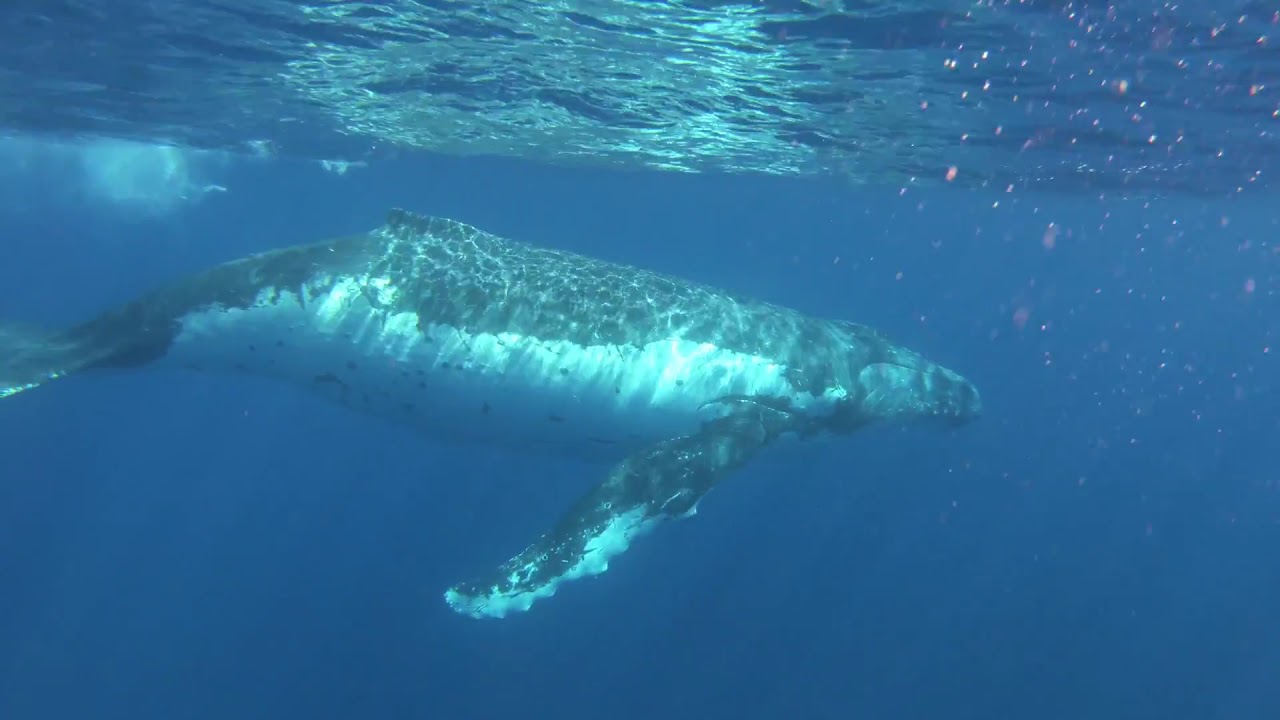This underwater photograph, likely captured by a scuba diver, features a large baleen whale swimming just beneath the ocean surface. The whale, one of the largest species, glides from left to right across the image. Its gray top and white underbelly are illuminated by scattered rays of sunlight penetrating the water, casting a spackled light effect on its body. The scene is set against a backdrop of rich, dark blues that transition to turquoise in the distance, with the visible water surface reflecting the sunlight and creating a wavy, shimmering effect. Sparse bubbles around the whale suggest it might have recently breached the surface. The photograph is devoid of other marine life, focusing entirely on this majestic mammal peacefully navigating the tranquil, clear blue sea. Little orange or red particles are faintly visible, possibly reflections from the diver's equipment.